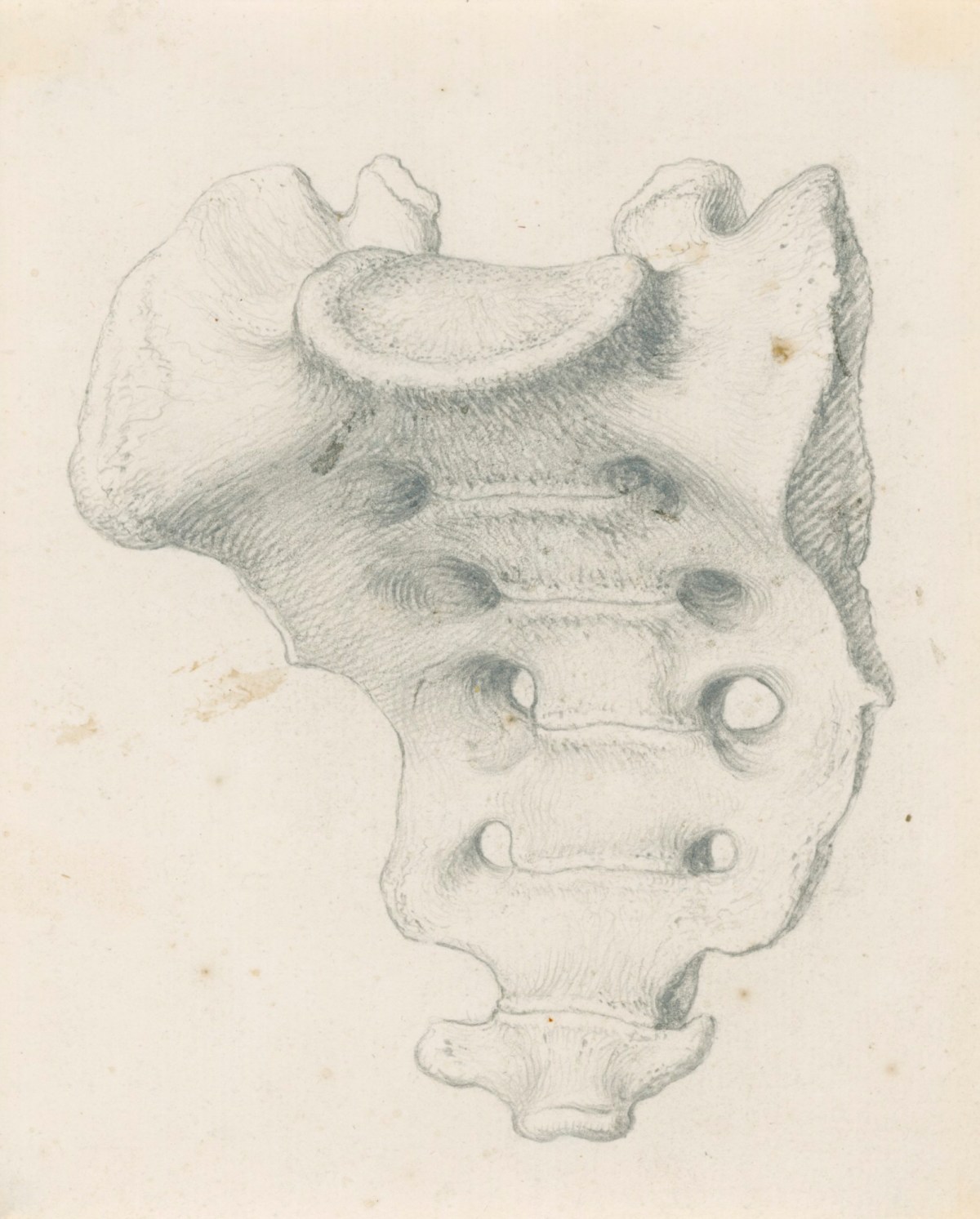This detailed illustration appears to be a meticulously crafted pencil sketch of an animal bone, potentially resembling vertebrae or a fossilized structure. The bone has a rectangular shape with an oval structure at the top, featuring multiple holes—specifically, four on each side for a total of eight. The top of the bone resembles a disc with slightly curved and elevated edges. The drawing is rendered on an old piece of paper, which is light pink with visible brown smears, water stains, and dust marks, suggesting its aged condition. The shading in the sketch is expertly done, highlighting the textures, shadows, and highlights, giving it a realistic and three-dimensional appearance.